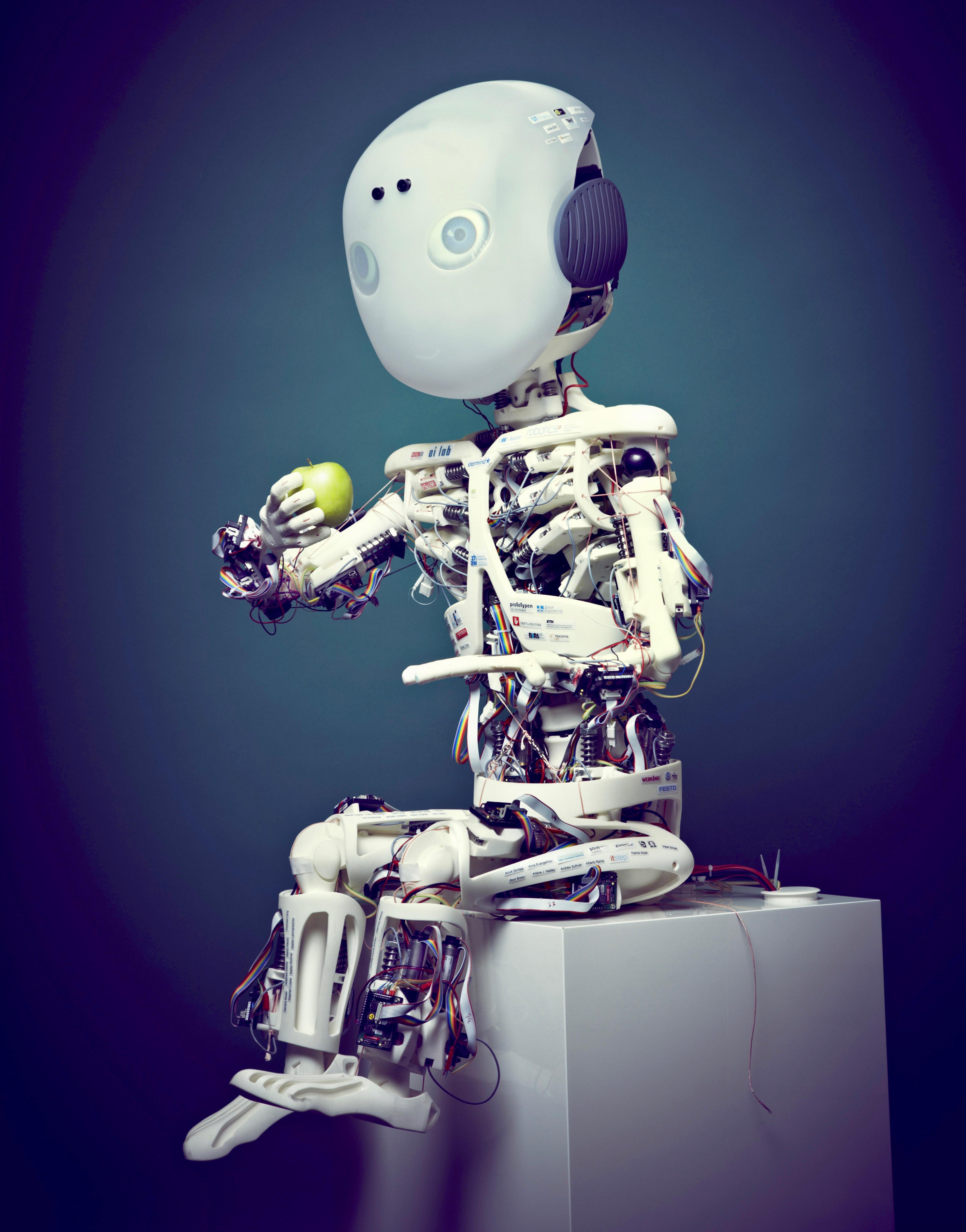The image depicts a highly detailed, complex white robot seated on a light gray cube set against a dark-to-light gradient blue background. The robot, composed predominantly of white plastic material, mimics human anatomical features with a torso, arms, legs, and feet. Its head, a half-dome of white plastic, features large, white eyes with blue detailing, above which are two black dots suggestive of additional sensors. Dark purple circles on the sides of the head resemble ears. The robot's right hand clutches a green apple as if preparing to take a bite, while the left hand extends forward, palm open. The sophisticated design also incorporates visible internal components such as black, blue, and red wires, enhancing the impression of intricate machinery at work.